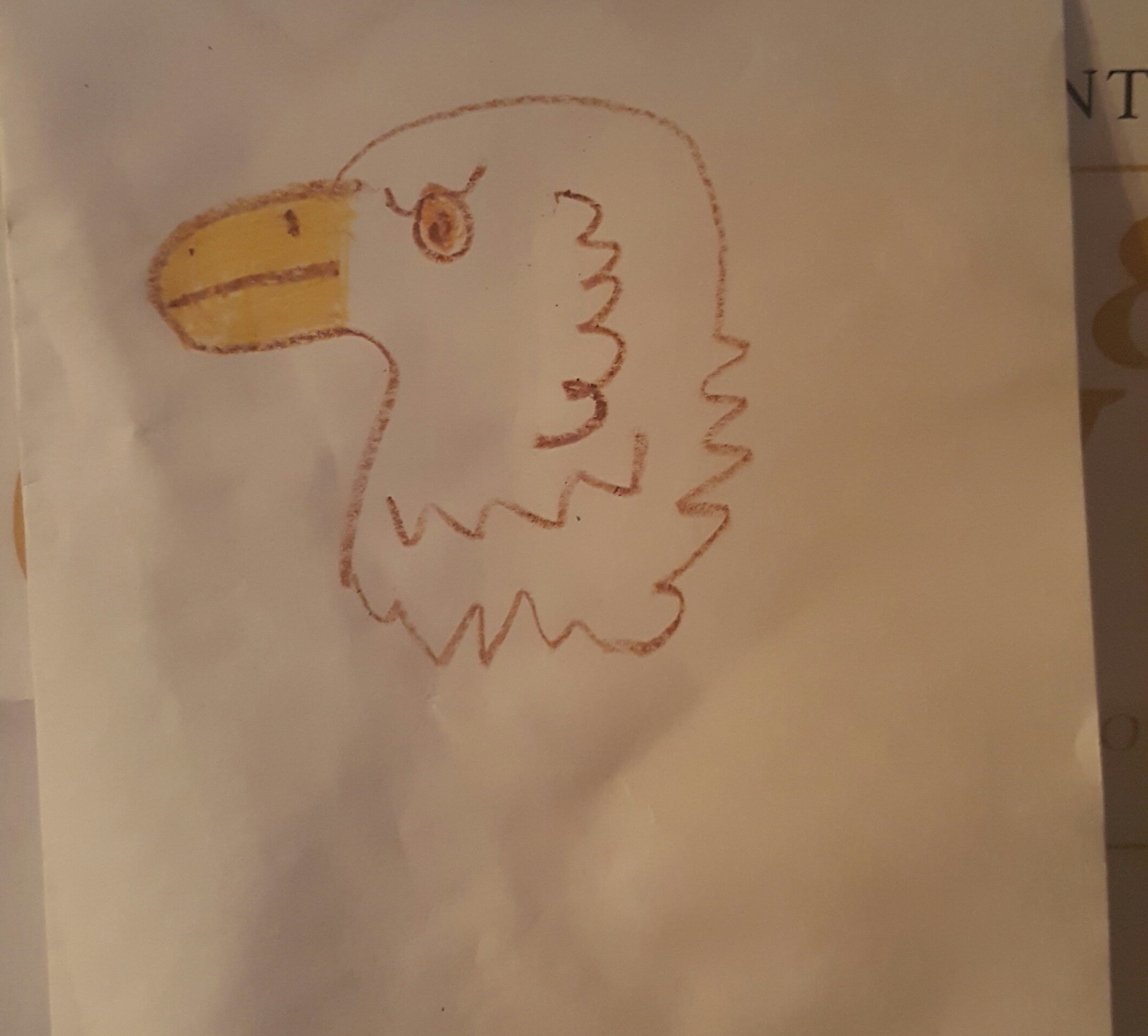This photo captures a detailed crayon drawing on a slightly crumpled white piece of paper, seemingly taped to a shadowed surface. The artwork presents a side profile of a well-proportioned bald eagle's head. The eagle’s head is outlined in one continuous brown marker line, while inside the neck area, there are squiggly lines indicating feather texture. The beak is colored in yellow with a defining horizontal brown line. The eye is a brown scribble that forms a circular shape. The overall simplicity of the drawing suggests it might be a child's work, despite its proportionate features. No shading is present, enhancing the focus on the clean, contour lines. The white paper has noticeable wrinkles, indicating it may have been slightly crumpled before being photographed.